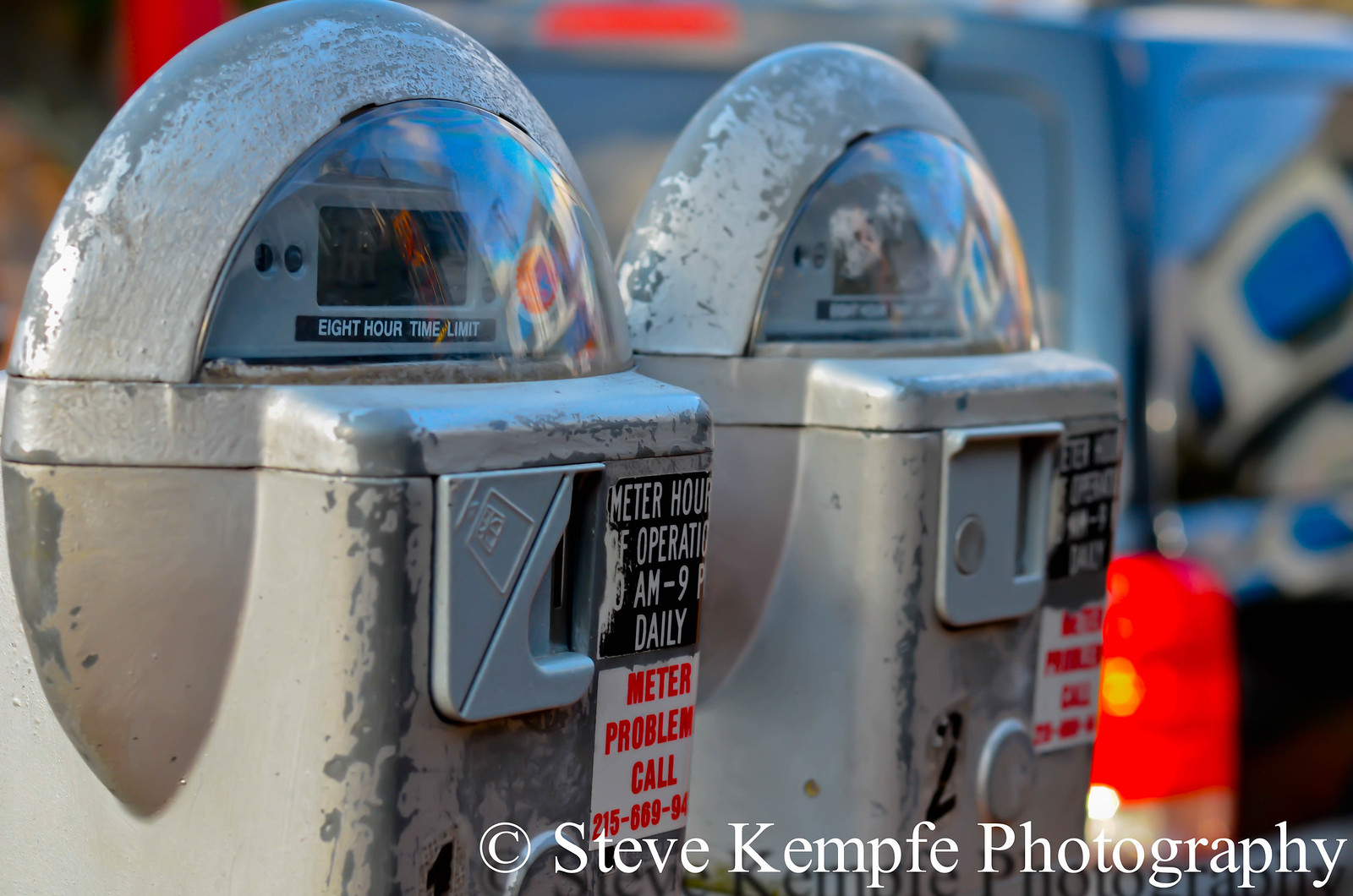This photograph offers a detailed close-up of two weathered parking meters set against an urban backdrop. The parking meters, both metallic in appearance with a faded gray coat revealing a darker gray primer beneath, display significant signs of wear with the paint chipping off substantially. Each meter features a dome at the top with white text indicating an "8-hour time limit," partially shielded by a glass covering. Below this, a small black bar and a cut-off message about the meter's hours of operation are visible. A prominent square ticket printer and stickers adorn the front of the meters. In addition to the main functional areas, there is a small square slot for coins and a barely discernible area indicating contact information for meter problems, suggesting the text might read something like, "meter problem call 215-669" followed by a partially cut-off number. The background of the image includes a glimpse of a large parked car and a partially visible red light, contributing to the bustling city scene. The photograph, taken during the day, has a distinctive stamp at the bottom corner that reads, "© Steve Kemp Photography."